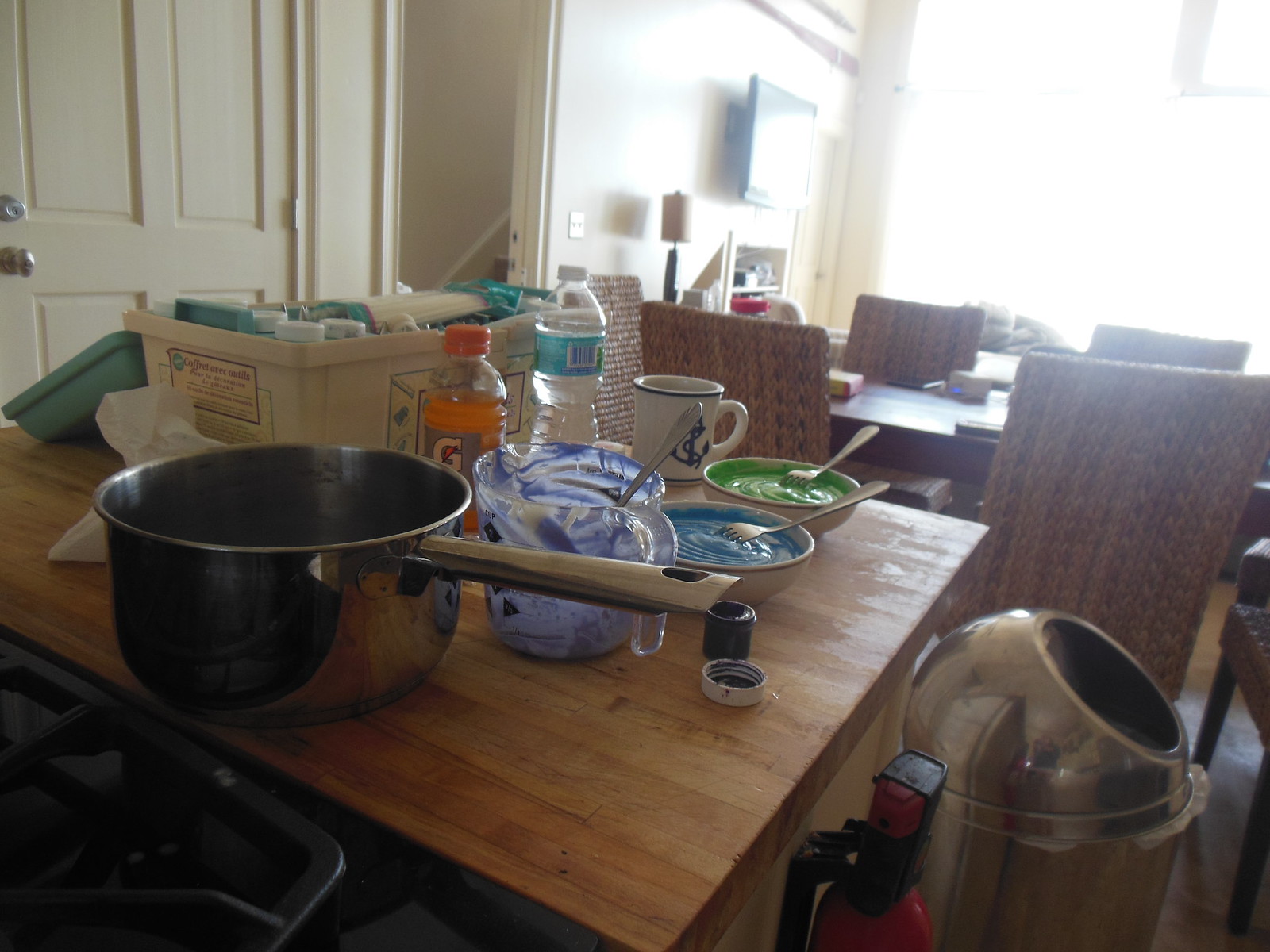In the image, a butcher block kitchen countertop is prominently featured. Positioned in the bottom right-hand corner, there is a stainless steel trash can with a rounded top and an open circular entry for disposing of waste. Mounted on the edge of the cabinet adjacent to the trash can is the top part of a visible fire extinguisher. Atop the butcher block countertop, numerous items are arranged: a pot of unknown contents, a measuring cup, and an open jar of food coloring. Accompanying these items are two bowls, one containing a blue mixture and the other a green mixture, each with a fork indicating recent stirring. Additionally, a bottle of water and an orange bottle of Gatorade are placed nearby. On the far edge of the counter, a toolbox or storage container is visible, likely filled with various cake decorating and baking materials, possibly including more jars of food coloring similar to the one seen in the foreground.